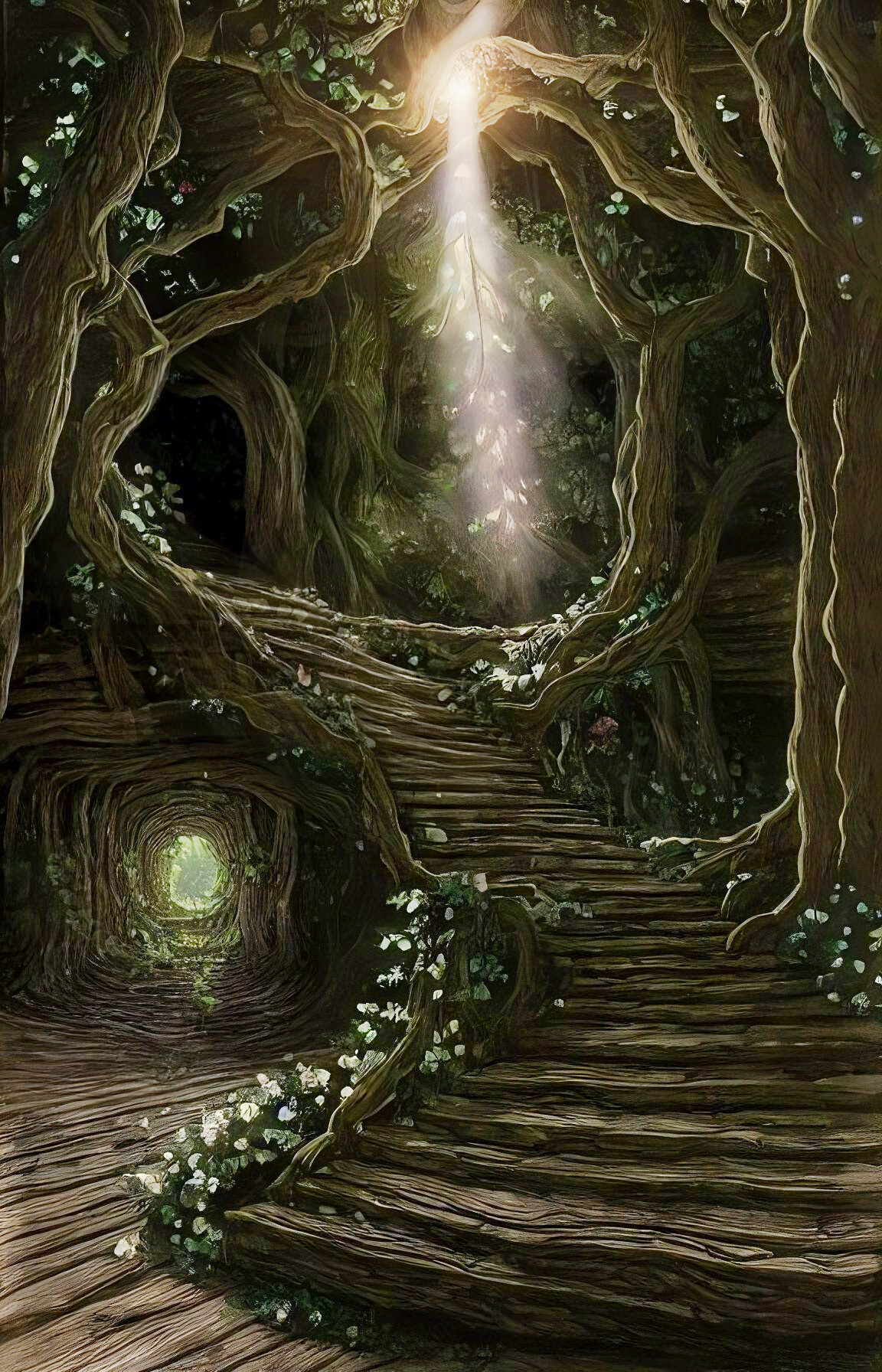This surrealist painting captures the mystical ambiance of a dense forest, bathed in a subtle cascade of sunlight. Large trees encircle the scene, their canopy allowing slivers of light to pierce through the dark forest floor. A unique, curved wooden stairway ascends from the forest ground, twisting upwards and to the left, culminating amidst the tree trunks. Adorning the sides of the steps are small, delicate white flowers, adding a touch of ethereal beauty. At the base of the stairs, wooden planks form a floor with a small hole, from which a soft glow emanates. On the left side, a tunnel-like structure with light seeping through its far end adds an intriguing element, leading out into the vivid greenery of the forest. The interplay of light and shadows, along with the intricate details of the branches and foliage, creates a mesmerizing and otherworldly feel.